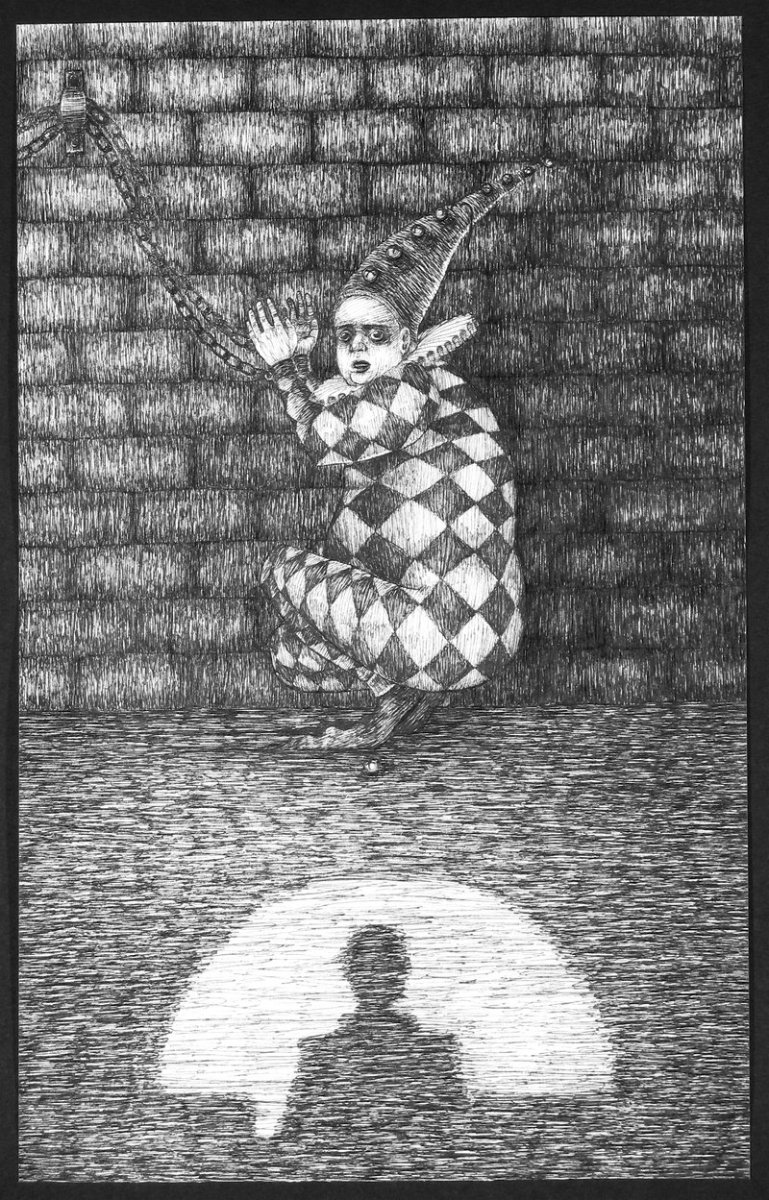The artwork is a detailed, black and white pencil or pen drawing, possibly a print, featuring a jester trapped in a dim dungeon. The jester, dressed in a traditional black and white checkered jumpsuit with a long, pointy hat adorned with bells and a ruffled neck collar, is chained by both wrists to a stone wall. He appears to be crouching or squatting, his hands raised to the level of his head as they are bound above him. An expression of fear marks his face. Long clown shoes complete his attire. The scene is further intensified by the stark lighting, suggesting an open door, casting the shadow of an obscured figure onto the dungeon floor. The atmosphere is eerie, devoid of any text or signature, heightening the mystery of the jester's plight.